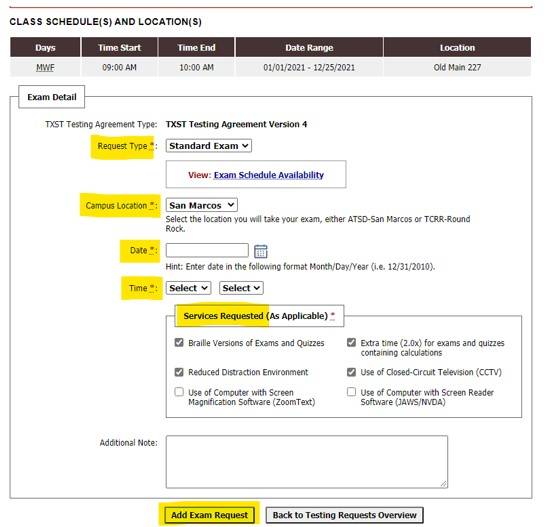This screenshot captures an interface displaying detailed information about a scheduled exam. The examination is confirmed as a standard exam, with a clear indication of the class schedule type at the top. Set to begin at 9 a.m. and conclude by 10 a.m., the exam falls within the date range from January 1, 2021, to December 12, 2021. It will be held at Old Main, room 227, which is likely a building located on the university's San Marcos campus.

Further details reveal that the exam adheres to Testing Agreement Version 4, though the specific date for the user's exam attempt has not been provided. Notably, the services requested for this exam include a braille version, extended time allowance up to twice the standard duration, the use of CCTV, and an environment with reduced distractions. There are no additional notes left for this request. The phrase "Add Exam Request" is also prominently highlighted in the screenshot, suggesting an option for scheduling or modifying exam requests.